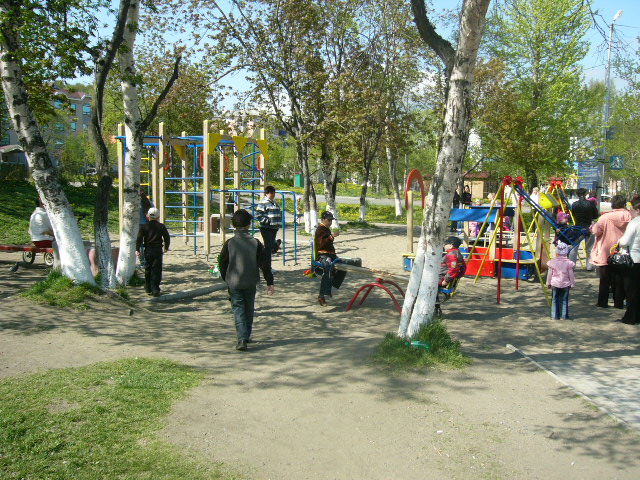This rectangular outdoor photograph captures a vibrant playground scene framed by several towering birch trees with their distinctive white, paper-like bark. In the playground area, a variety of brightly colored playground equipment is scattered around, including a jungle gym, multiple swing sets, and a seesaw situated centrally. The playground area itself is divided into a sandy section and a worn-down grassy area, where patches of grass are interspersed with dirt from heavy use. 

Children and adults are dispersed throughout, some climbing on the jungle gym, others enjoying the swings, and a few sitting on a bench to the left. The adults and kids, many of whom are clad in jackets, hoodies, and hats, suggest a chilly day. To the right of the image, a paved pathway leads up to the sandy playground section. 

In the background, beyond the playground, a road is visible with buildings and additional trees lining the horizon. The sky, dotted with clouds, peeks through the branches, adding a touch of serenity to the lively ambiance.